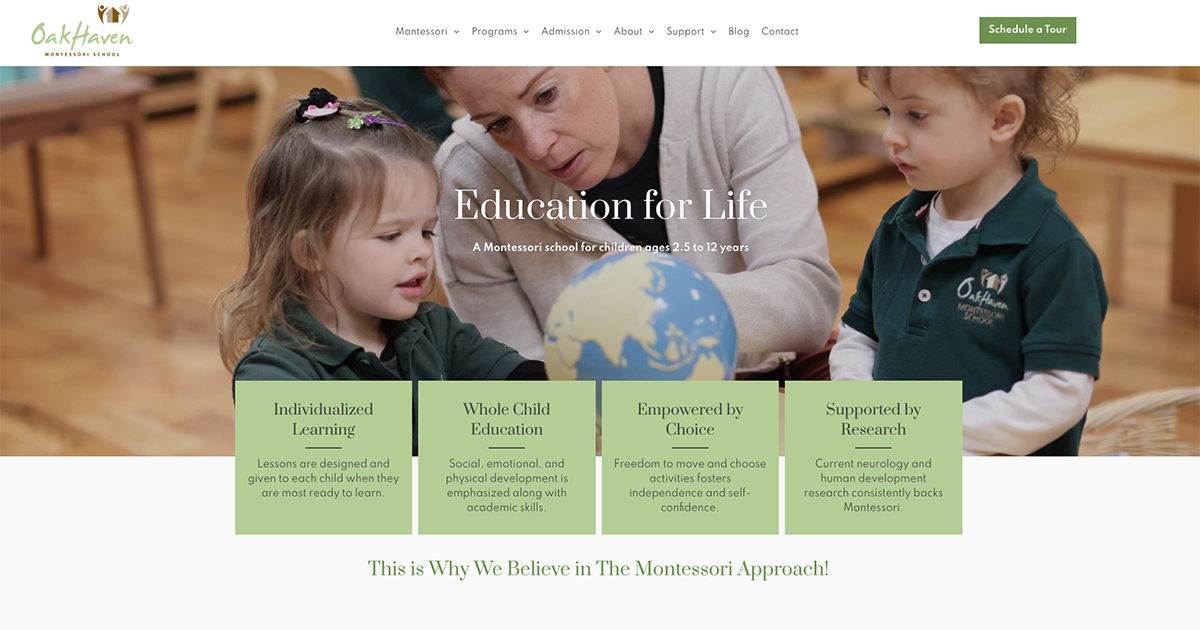This image is a screenshot from the webpage of O'Kaven Montessori School. The school's name, "O'Kaven Montessori School," is prominently displayed in green text in the top left corner. The top navigation bar, which is white, features several drop-down menus including "Montessori," "Programs & Mission," "About," "Support," "Blog," and "Contact." On the right side of this bar, there is a green button labeled "Schedule a Tour."

Below this bar, an image depicts a teacher engaging with two young children, who appear to be toddlers. The children are dressed in green uniforms that bear the school's name. The title underneath the image reads, "Education for Life: A Montessori School for Children Ages 2.5 to 12 Years."

Beneath the title are four green informational boxes. The first box, titled "Individualized Learning," states, "Lessons are designed and given to each child when they are most ready to learn." The second box, "Whole Child Education," notes that "Social, emotional, and physical development is emphasized along with academic skills." The third box, "Empowered by Choice," highlights that "Freedom to move and choose activities fosters independence and self-confidence." The fourth and final box, "Supported by Research," conveys that "Current neurology and human development research consistently backs Montessori."

At the bottom of the image, green text declares, "This is why we believe in a Montessori approach!"